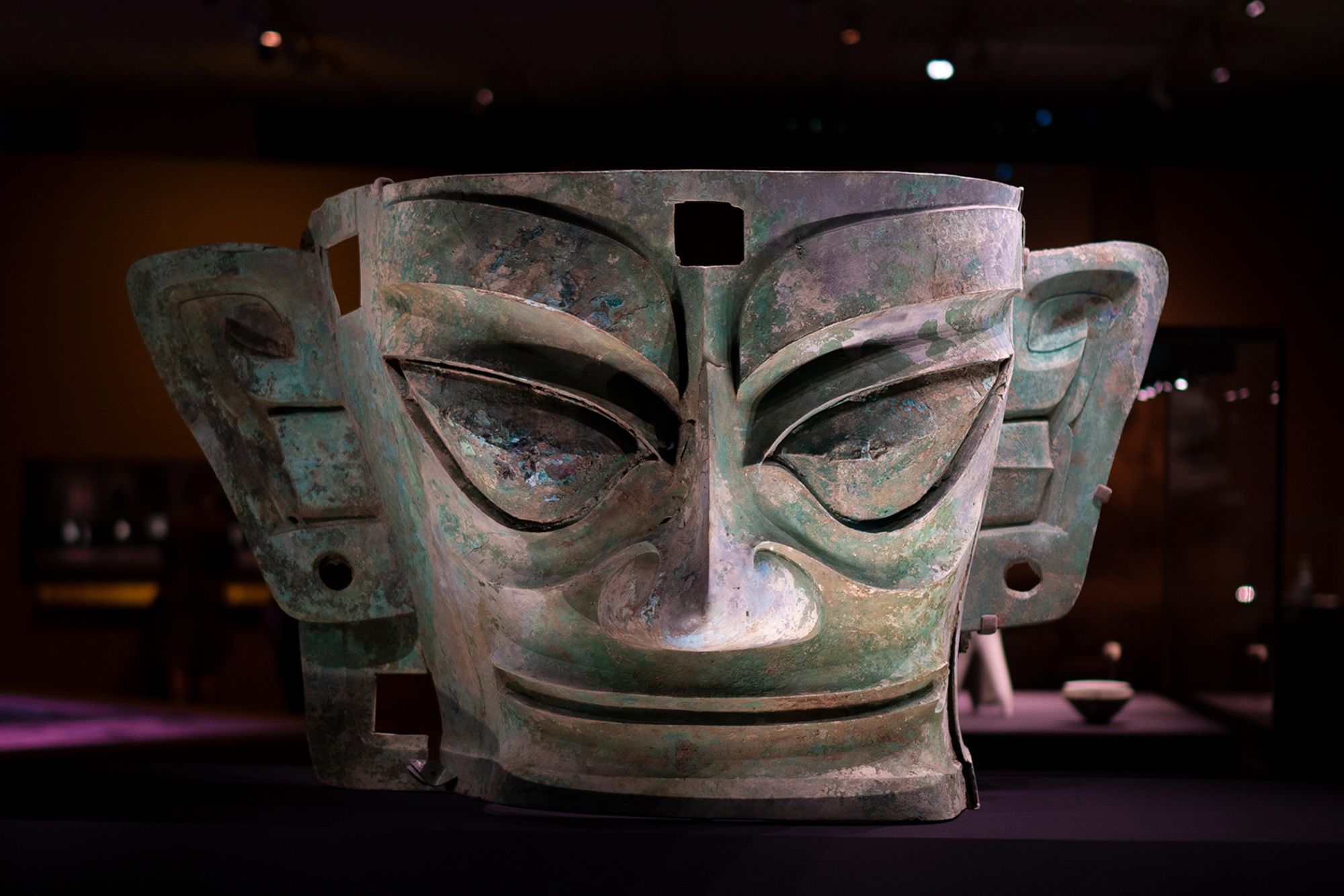This detailed description captures the essence of the large metal sculpture depicted in the image:

---

The photograph showcases a giant metal sculpture of a head, prominently displayed against a dark background with hints of purple light from below, likely in a museum setting. The sculpture, which exudes a primitive, tribal design, is characterized by its aged patina of varying shades of green, brown, and rusted metal. 

The face of the sculpture is front-facing, illuminated brightly to reveal intricate details. Its eyes are distinctive, with pointed upper corners and rounded lower edges, creating a wide-eyed expression. The bulging eyeballs and the weather-beaten, wrinkled texture around them suggest an antiquated, weathered artifact. Metal eyebrows angle slightly downward toward the center, just above a sharp-ridged nose with slightly flared nostrils.

Below the sharp nose is a thin, black curved line representing the mouth, giving a subtle smile. A thin ledge forms the chin, adding to the defined facial structure. Noteworthy is the rectangular hole cut out on the forehead and the square cut just above it, adding to the uniqueness of the piece.

The sculpture also has large, protruding rectangular ears with multiple sections separated by lines and pierced holes at the lobes, suggesting they could be used as handles. The ears' design and their pristine white color provide a striking contrast to the rest of the face.

Overall, this detailed and evocative sculpture stands as a focal point on a dull purplish carpet, surrounded by blurred, indistinct museum artifacts visible just in the background. The interplay of shadow and light amplifies the intricate textures and timeworn appearance of this fascinating art piece.